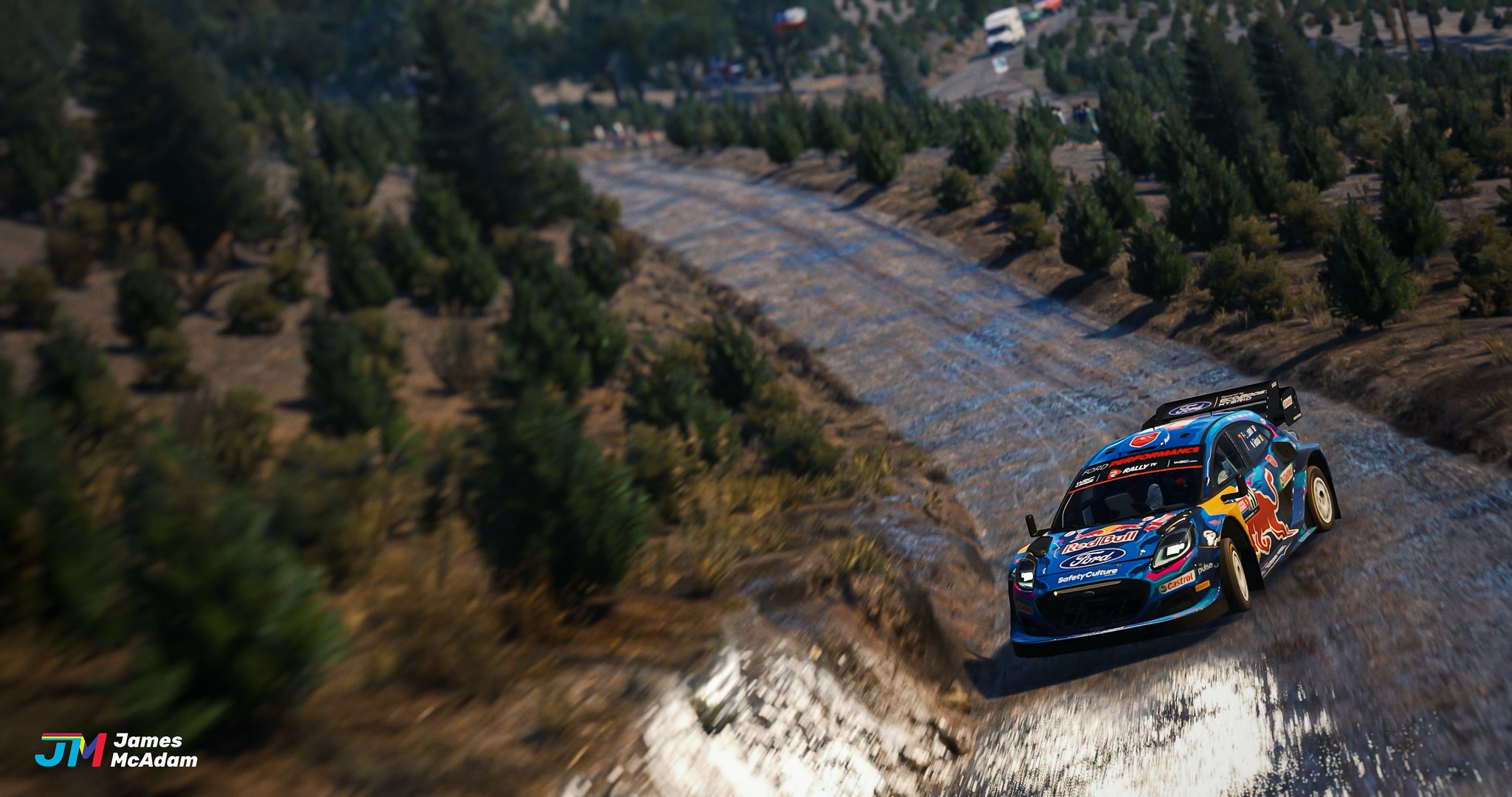The photo captures a blue race car speeding along a practice track. The image is slightly blurry, emphasizing the car's high velocity. The race car is adorned with multiple sponsor decals, including prominent Ford logos and what appears to be a camel graphic on one side. It features black tires and a black rear spoiler. The road ahead of the car has white patches, which could be snow or reflections on wet pavement. Flanking the track are sections of brown dirt lined with small, evergreen trees, adding a natural contrast to the scene. In the bottom left corner, the photo is credited to JM James McAdams, possibly the photographer's signature.